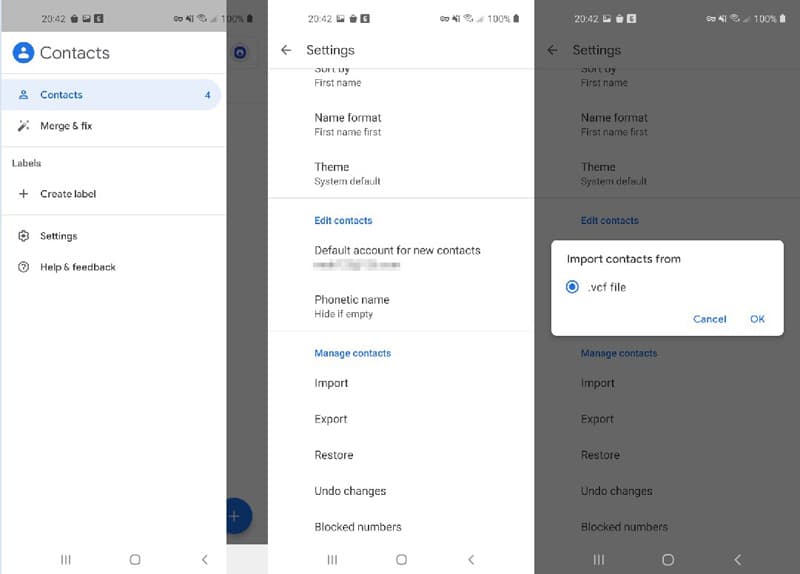The series comprises three sequential screenshots displaying a contacts management interface on a mobile device.

### Screenshot 1:
The top of the first screenshot shows a status bar with a gray timestamp reading "20:42" and a Wi-Fi icon. Below, a white menu panel features blue and gray text. The header reads "Contacts" next to a blue circle icon. The menu contains the following items:
- "Contacts (4)" with a small person icon
- "Merge and fix" with a magic wand icon
- "Labels" section with a "Create label" option, accompanied by a plus sign icon
- "Settings" represented by a cogwheel icon
- "Help and feedback" marked by a circle with a question mark icon

At the bottom of the screenshot, navigation icons include three horizontal lines, a square, and a back arrow.

### Screenshot 2:
The second screenshot, also time-stamped "20:42," maintains the same status icons as the first. Below, the white background with green and blue text reads "Settings." Key settings items listed include:
- "Name format: First name first"
- "Theme: System default"
- "Edit contacts"
- "Default account for new contacts" (followed by a blurred out email address or phone number)
- "Phonetic name: Hide if empty"
- "Manage contacts" with options to "Import," "Export," "Restore," "Undo changes," and "Block numbers"

The bottom navigation icons, similar to the first screenshot, consist of three horizontal lines, a square, and a back arrow.

### Screenshot 3:
The third screenshot, featuring a slightly grayed-out overlay, retains the same top status bar with the "20:42" timestamp and identical icons. The primary content shows the "Settings" menu items from the second screenshot. In addition, a white pop-up box appears with black text stating "Import contacts from," followed by a blue circle labeled ".bcf file". Two blue buttons at the bottom of the pop-up offer the options "Cancel" and "OK."

As in the previous screenshots, the bottom navigation icons include three horizontal lines, a square, and a back arrow.